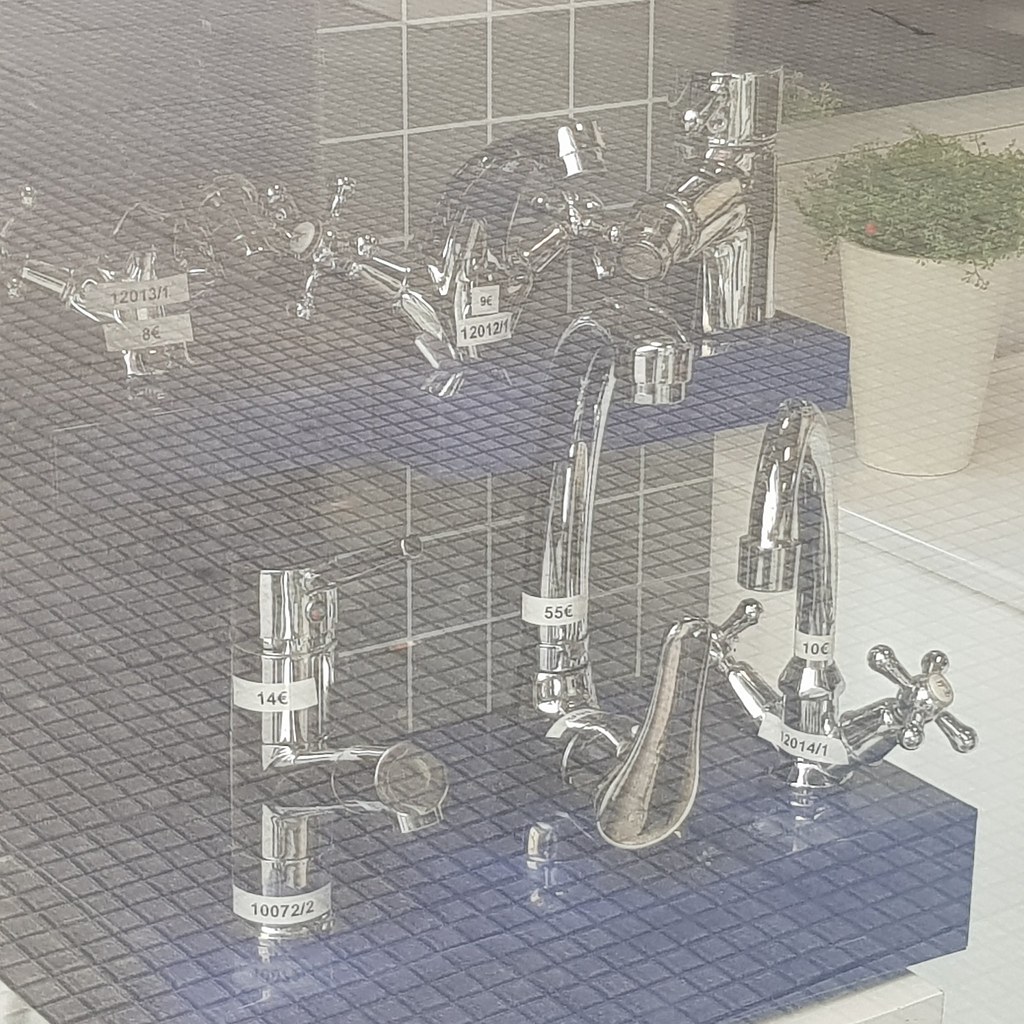This photograph, taken through a wire mesh or screen, showcases a display of six unique chrome faucets meticulously arranged on blue tiled shelves with a matching gray tile backsplash. The composition includes faucets of varying configurations – some with handles on the side, one with a handle on top, and another with a handle underneath, demonstrating a variety of contemporary designs. Notably, one faucet features a diagonal on/off mechanism with hot and cold controls jutting out uniquely, while another boasts a tall neck with a front-facing handle. Each faucet is marked with a price sticker in euros, indicating they are for sale, possibly within a store setting. Adjacent to the faucet display is a small white planter with greenery, providing a touch of nature amidst the modern fixtures. The photograph's hazy quality, likely due to the intervening mesh, adds a subtle artistic filter to the scene.